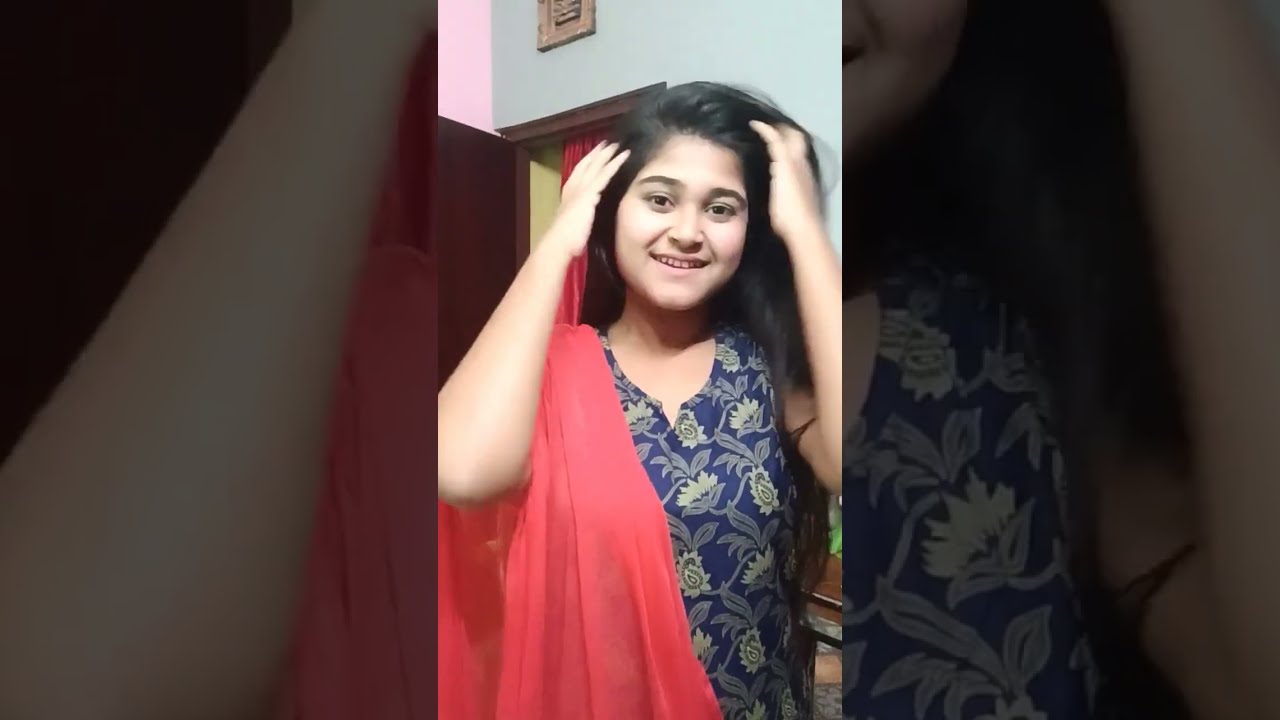The image is divided into three segments with the left and right segments darkened by some filter or film. In the center segment, the main focus is a young girl, likely between 11 and 12 years old, who is possibly of Indian or Middle Eastern descent. She has long, shiny black hair and dark eyes and is running her fingers through her hair. She is smiling, revealing the top row of her teeth, and looking directly at the camera. The girl is wearing a blue v-neck dress adorned with yellow floral patterns and has a red sash draped over her right shoulder. The background features a room with different colored walls—light green and pink—as well as a dark wooden doorway frame with a beige-brown vent above it. Through the doorway, part of a pale green wall and a red curtain can be seen.